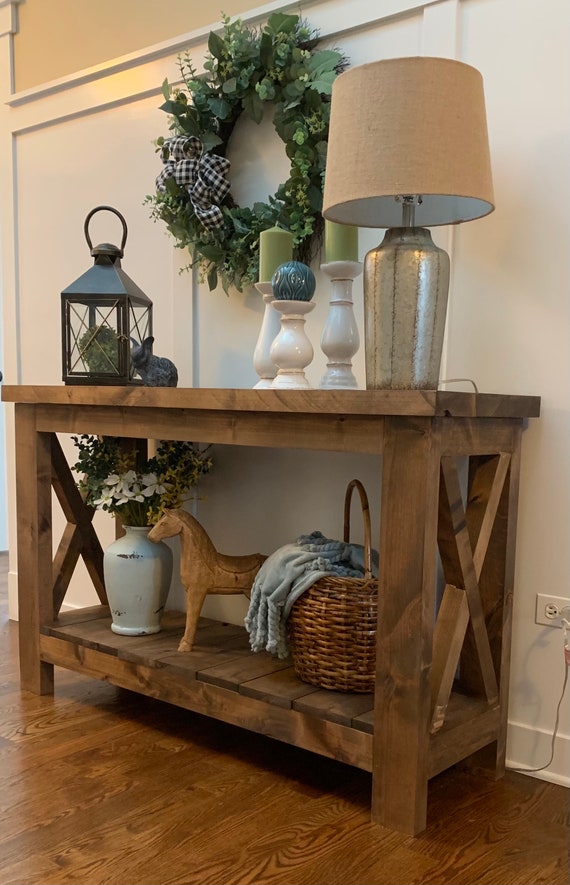This color photograph captures a close-up of a small farmhouse-style wooden entryway table with an x-shaped design on each side, showcasing intricate details that define its rustic charm. The table features two shelves and sits on polished hardwood floors against a pristine white shiplap wall.

On the bottom shelf, a wicker basket with a blanket partially draped over the edge sits alongside a carved wooden horse and a weathered white metal vase holding white flowers and eucalyptus. These items are complemented by the natural wood tones and the greenery, adding a cozy and inviting feel to the space.

The top shelf is adorned with a silver ceramic lamp with a tan shade positioned on the right-hand side, its cord trailing discreetly behind the table. Next to the lamp are three white ceramic candlesticks; two hold green pillar candles, while the third one supports a small blue ball candle. To the left side of the top shelf, a black metal lantern encases a moss ball, adding a touch of whimsy beside a small black figurine of a rabbit, further enhancing the rustic aesthetic.

Above this thoughtfully arranged table, a vibrant green wreath adorned with a blue and white checkered bow is mounted on the shiplap wall, bringing a cohesive and charming touch to the farmhouse-style decor.